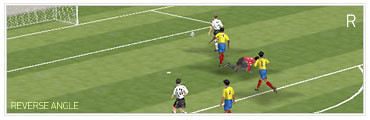This vibrant, wide-aspect color image captures an intense moment on a meticulously maintained football pitch. The grass is freshly mowed in alternating light and dark green stripes, giving a beautiful contrast. At the lower-left corner, there's white text, though it's not entirely legible. The scene is viewed from a reverse angle, focusing on the players and the field's details.

In the upper left, a white goalpost stands prominently, with a clearly marked white rectangle beneath it, indicating the goal area. White lines crisply outline various zones on the pitch, enhancing the field's structure.

At the center of the image, the action unfolds. Players in yellow jerseys and blue shorts are in motion, with one of them having just launched the ball into the air, which hovers over his head. Amidst them, a player in a white jersey and black shorts stands out, possibly preparing to intercept or redirect the ball. On the ground, another player wearing a red jersey and black shorts appears to have fallen or slid in an effortful play.

In the upper right corner, the letter "R" is visibly marked in white, possibly part of a larger text or a logo that is partially cropped out of the frame. This dynamic and detailed image vividly captures the energy and spirit of a football game.